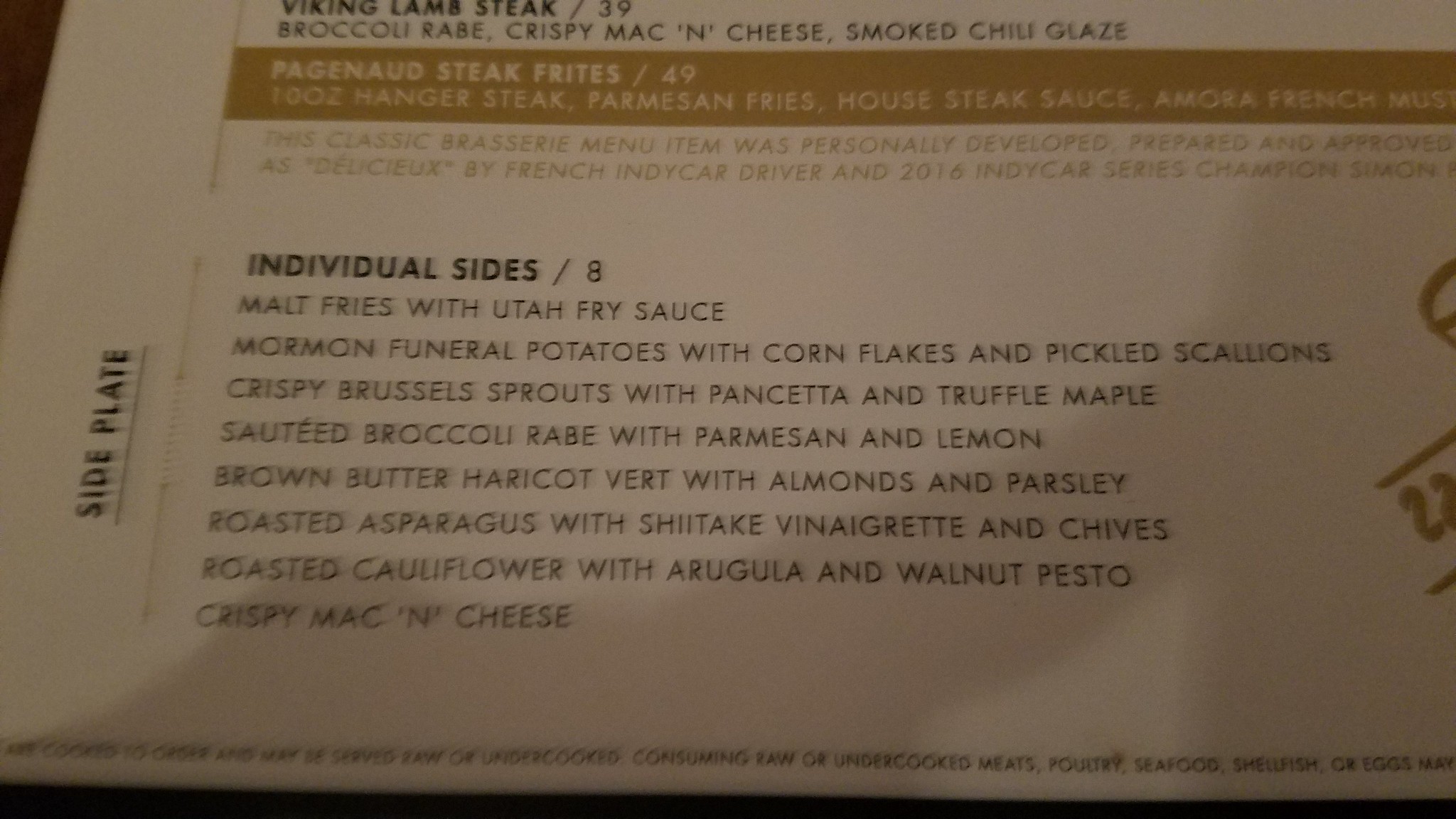This image features a restaurant menu printed on white paper with black text. The menu, although somewhat blurred, predominantly showcases a section dedicated to individual side dishes, all priced at $8 each. The section header "Individual Sides" is presented in bold font. The specific sides listed include:

1. Malt Fries with Utah Fry Sauce
2. Mormon Funeral Potatoes with Cornflakes and Pickled Scallions
3. Crispy Brussel Sprouts with Pancetta and Truffle Maple
4. Sautéed Broccoli Rabe with Parmesan and Lemon
5. Ground Butter Halicot Gherk with Almonds and Parsley
6. Roasted Asparagus with Chitay Vinaigrette and Chives
7. Roasted Cauliflower with Arugula and Walnut Pesto
8. Crispy Mac and Cheese

Above the individual sides section, there appear to be listings for main courses, though these are difficult to read due to the blurriness of the image. The menu's color scheme involves a primarily white background with beige accents, offering a sophisticated presentation. Overall, the variety of unique and intriguing side dishes suggests that this is a restaurant with a creative and unusual culinary approach.